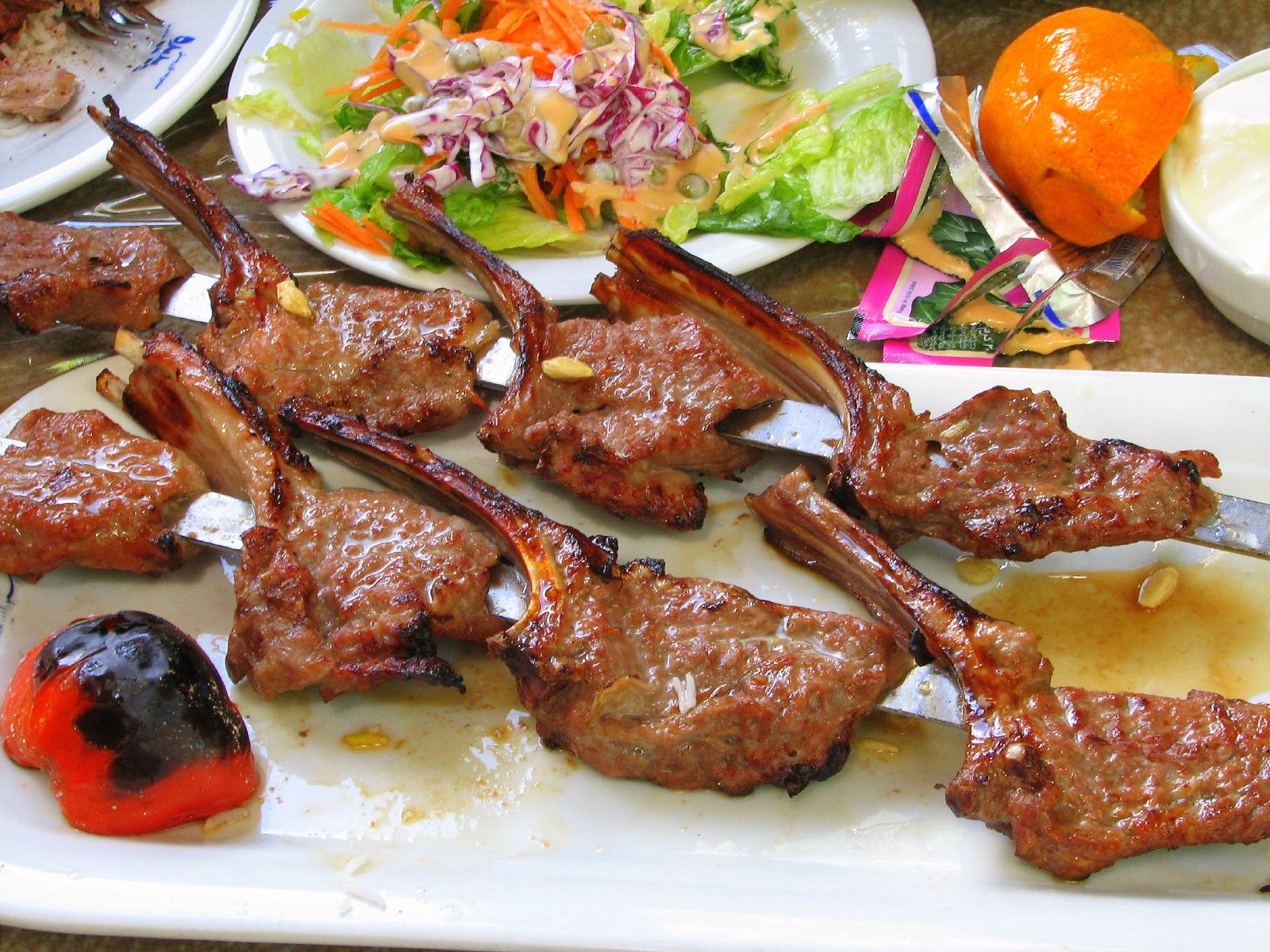The photograph showcases a detailed display of food on a brown surface, likely a table. Central to the image is a long, rectangular white ceramic platter containing four chop-style cuts of cooked meat, potentially pork or lamb. Each piece is pierced by a silver implement resembling flat skewers, with juices and a brown sauce dripping off the meat. Surrounding the chops are lemon seeds and a half-charred red bell pepper.

Adjacent to the meat platter, towards the top center, there's a white circular plate filled with a vibrant salad. The salad is composed of shredded carrots, cabbage, and green lettuce, lightly coated with what appears to be a Thousand Island dressing. In front of this plate is a tangerine peel, adding a pop of orange color. 

In the upper right corner, partially cut off, is a white bowl containing a creamy white substance, possibly a sauce or dip. The intricate array of textures and colors, from the charred and saucy meat to the fresh green salad and bright orange peel, creates a rich and inviting culinary presentation.